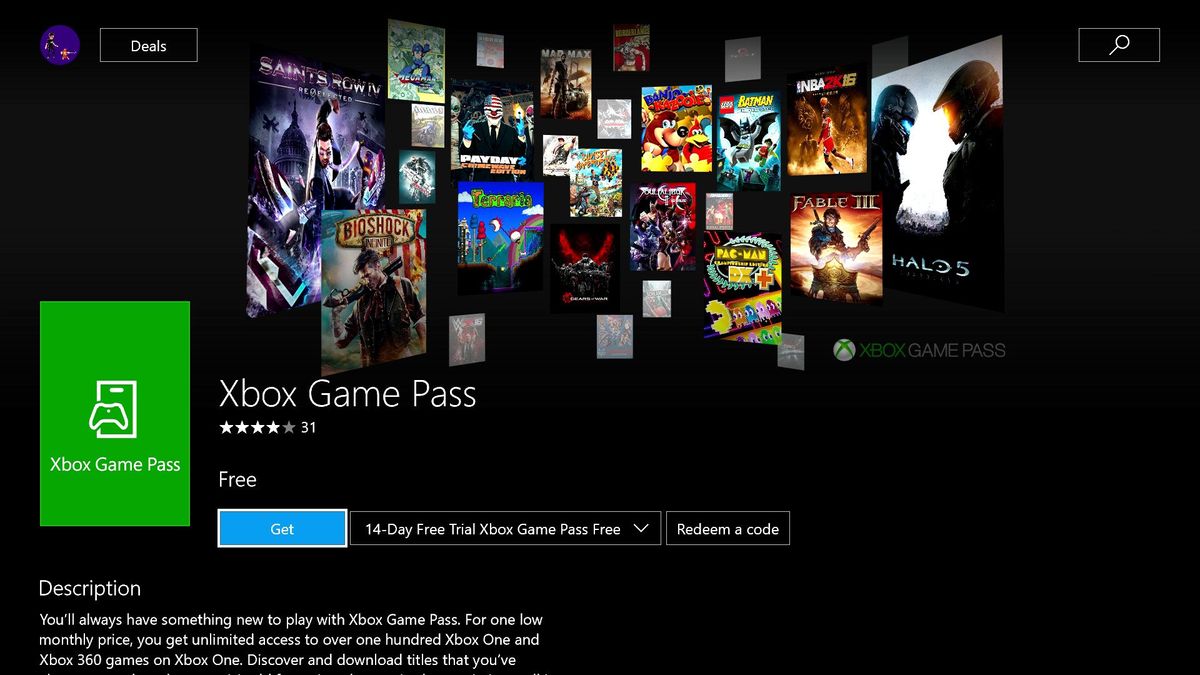The image is a high-resolution screenshot of the Xbox Game Pass website, displayed on a rectangular, horizontal screen with a sleek, black background. In the center of the image, a vibrant gallery of video game covers is prominently showcased, each illuminated against the dark backdrop. To the right, a captivating image of two armored soldiers represents "Halo 5." On the left side, a menacing character wielding a gun is depicted, indicating "Bioshock."

Further to the right, a dynamic shot of a Lego Batman stands out, while just below it, a striking image from "NBA 2K16" features a player, clad in a red uniform, performing a slam dunk. Nestled beneath these images, a prominent, vertical green rectangle grabs attention, emblazoned with the Xbox Game Pass logo.

Adjacent to the green rectangle, white text reads "Xbox Game Pass" with a four-star rating underneath, along with the word “Free.” Nearby, a distinct blue button marked "Get" invites viewers to click. Directly below, it offers a "14-day free trial Xbox Game Pass free" with an option to "Redeem a code." The bottom left corner of the screen contains some small, less legible text.